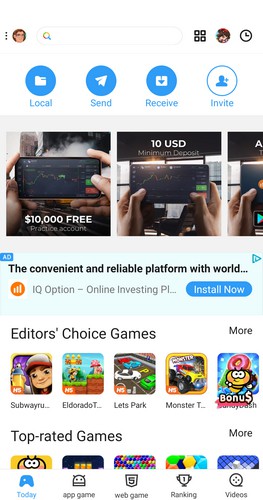**Caption:**

A mobile app interface displaying a well-organized layout, seemingly tailored for app management and investment tracking. At the top of the screen, there is a navigation bar featuring three vertical dots on the left, followed by a user profile image, a search bar, and an icon consisting of four small squares forming a larger square. Adjacent to these, another user profile picture is visible along with a set timer.

Centrally positioned at the top, four buttons are aligned horizontally. The first three buttons are blue with white icons, labeled "Local," "Send," and "Receive." The fourth button is white with a blue icon, labeled "Invite."

Below these buttons is an advertisement showcasing three images of an individual using their phone, presumably engaging with the stock market. The text on the ad promises a $10,000 free practice account with a 10 USD minimum deposit, though the rest of the text is cut off.

Further down, another advertisement appears with a blue "Ad" indicator. It advertises a "convenient and reliable platform" for investing, branded as "IQ caption," and prompts users to "install now."

The interface continues with a section titled "Editor's Choice Games," featuring popular games such as Subway Surfer, El Dorado, Let's Park, Monster, and Bonus. A button labeled "More" offers additional choices. Lastly, the "Top Rated Games" section presents a further selection of highly rated games on the platform.